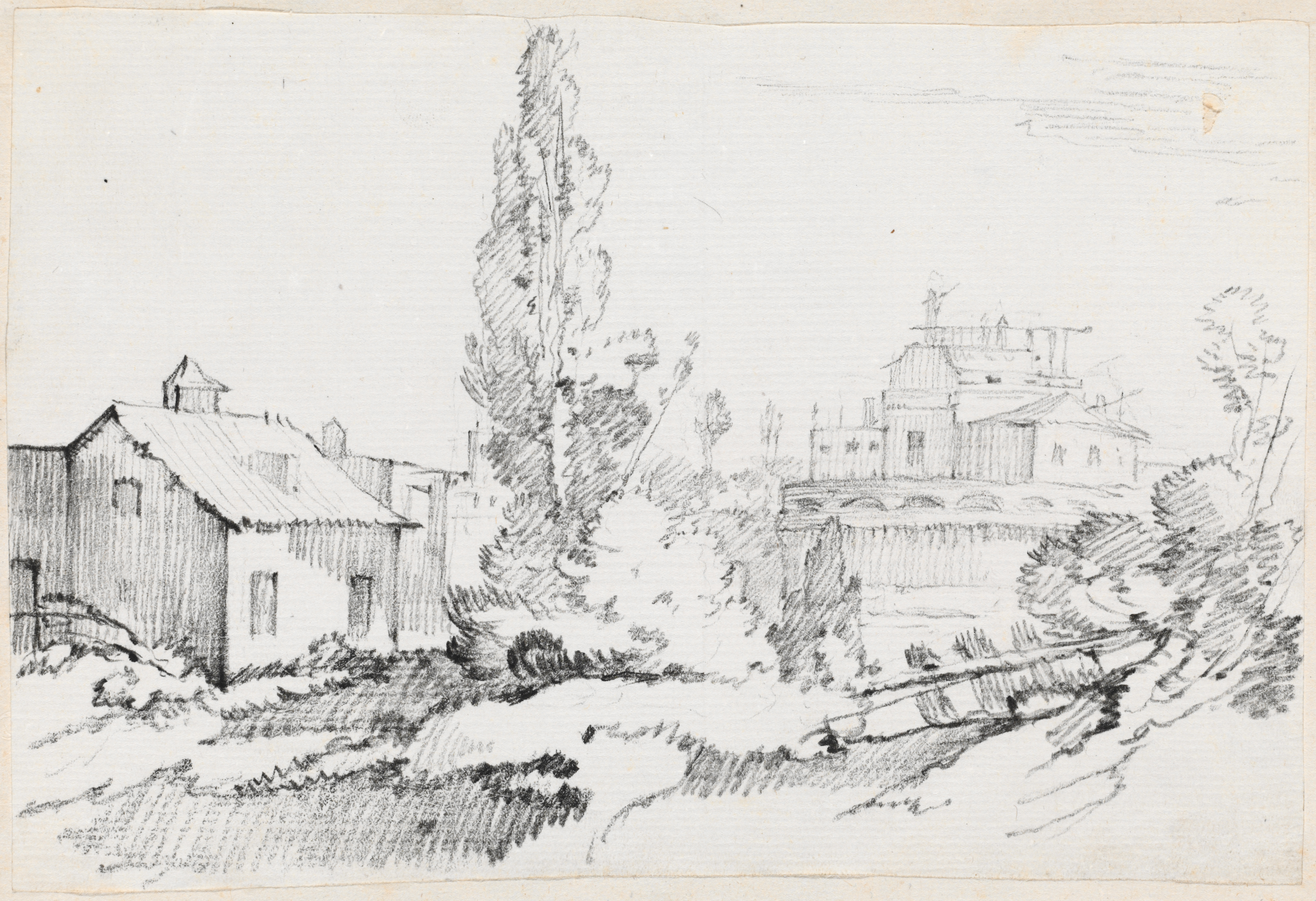The image is a black and white drawing, seemingly rendered with a regular pencil. This detailed sketch features a country setting with multiple structures and elements of nature. On the left side, there is a two-story farmhouse characterized by two windows on the bottom floor, one window on the top floor, and a chimney. The farmhouse also showcases an arched roof. In the foreground and to the right of the farmhouse stands a tall tree, accompanied by several bushes and other patches of vegetation.

Further off in the distance, on the right side of the drawing, a larger building looms, which some might interpret as a castle or possibly a church due to its imposing size and arched entrance. This larger structure has varying heights, suggesting an intricate architectural design. The background features additional smaller buildings with arched roofs, adding depth to the scene. The sloping ground in the foreground gradually descends towards the distant larger structure, where more foliage and tall trees are observed, completing the idyllic country landscape depicted in this monochromatic artwork.